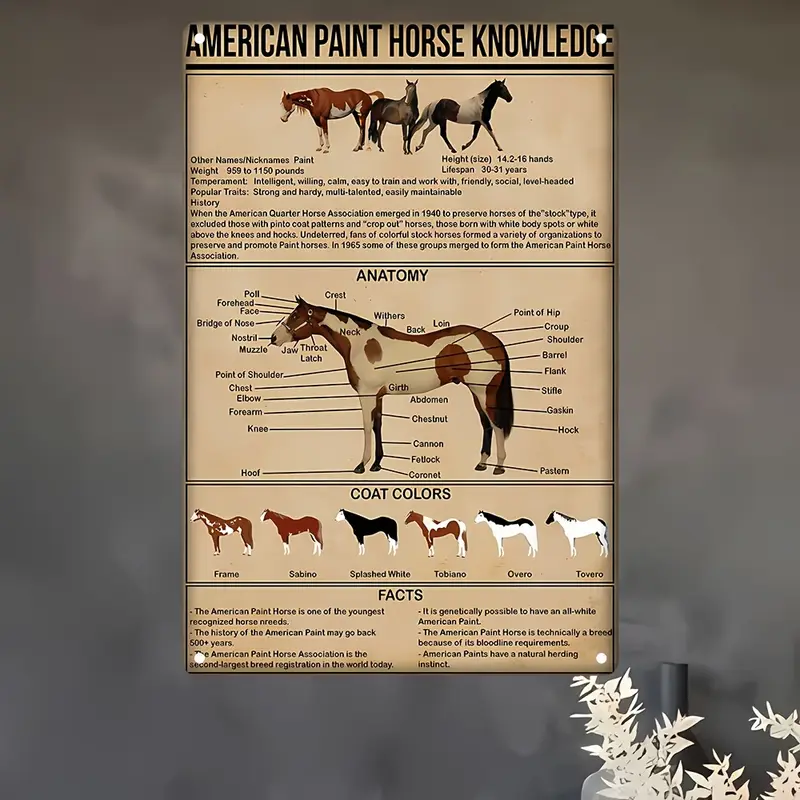The poster, titled "American Paint Horse Knowledge," is a comprehensive visual guide on the American Paint Horse breed. At the top, the title is prominently displayed. Below it are images of three horses with accompanying text in small print, describing them. The horses showcased include a brown and white one, a black one, and a black and white spotted one. 

Central to the poster is a detailed anatomical diagram of a brown and white horse, labeled "ANATOMY" in all capital letters. The diagram features lines pointing to various parts of the horse's body such as the knee, pastern, fetlock, cannon, chestnut, and abdomen, offering a thorough understanding of its structure.

At the bottom of the poster, under a set of double black lines, there is a section titled "COAT COLORS," providing additional information on the various hues and patterns found in the breed.